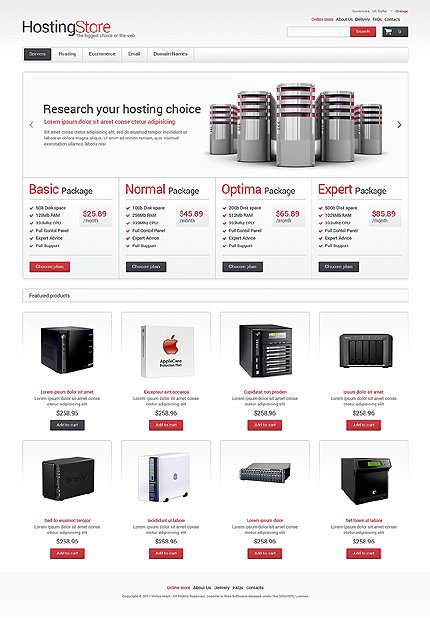This is a screenshot of a mock-up website called "Hosting Store," showcasing a detailed preview of a dummy design layout. The background features a gradient transitioning from light gray at the top to white near the bottom, which provides a visually appealing backdrop for the content. The bottom of the page includes a solid gray footer bar.

The top portion of the website highlights various hosting packages, each accompanied by a list of specifications marked with red checkmarks and described in black text. A red price tag within a gray box is displayed to the right of the list. The buttons, which appear to represent a selection action (likely "Choose"), come in two color schemes: white text on a red background and white text on a black background.

The overall color scheme of the site prominently utilizes red, black, and white. The individual product listings below the hosting packages feature product names in bold red text and descriptions in standard black text, all using placeholder text (Lorem Ipsum) indicating that this is not a real website.

Eight products are presented in two rows of four, reflecting the four different hosting packages displayed above. The pricing for these packages ranges from $25.89 to $85.89 per month. This design helps visualize how different elements and color schemes might look on an actual website.